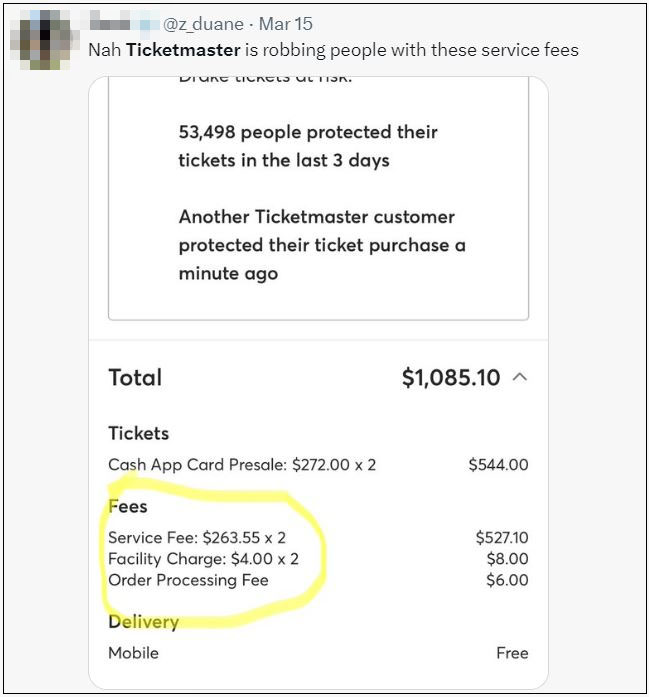Light gray background screenshot of a social media post with a blurred profile image and the tag "@Z_DUANE." The post date is March 15th with the comment "NAH" and then a bold "Ticketmaster" followed by "is robbing people with these service fees." 

A white rectangle with a black text overlay states "53,498 people protected their tickets in the last three days" and "Another Ticketmaster customer protected their ticket purchase a minute ago," with a thin gray line below.

The pricing information is displayed as follows:
- **Total:** $1,085.10
- **Ticket cost:** $272.00 (×2 = $554.00)
- **Fees:** 
  - Service Fee: $263.55 (×2)
  - Facility Charge: $4.00 (×2)
  - Order Processing: $527.10
  - Total additional fees: $8.00 + $6.00
- **Mobile delivery:** Free

The fees section circled in yellow highlights the extensive service charges applied by Ticketmaster, criticizing the high costs.